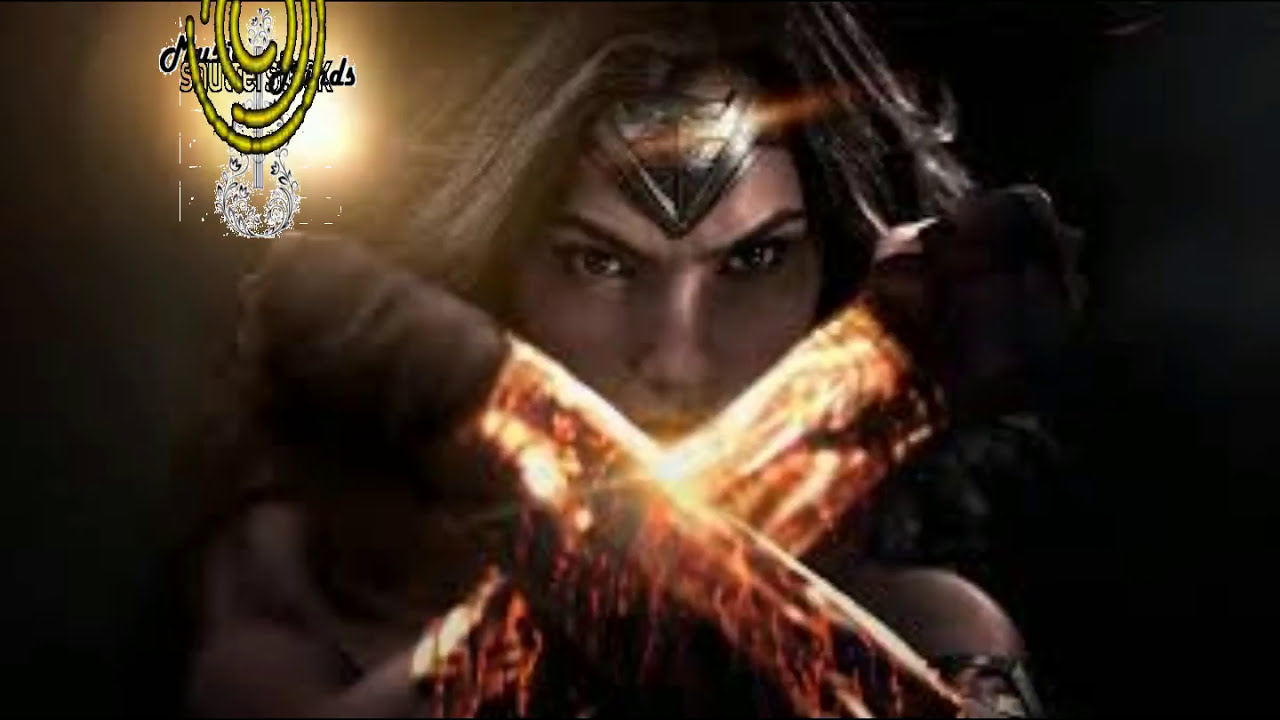The image depicts a fierce warrior woman with intense, fiery eyes, radiating determination as she stands with her arms crossed in front of her. Her forearms, adorned with glowing, fire-colored armor in hues of orange, yellow, and red, appear to be molten and ablaze, casting an eerie, intense glow. She is clad in dark gloves and body armor, and wears a metal visor crown with a triangular design across her forehead. Her thick, wavy, dark brown hair flows behind her, contrasting sharply with the dark, shadowy background that envelops her. The scene is dramatically lit, emphasizing her fiery forearms and the cold metal headgear she dons, making her look powerful and ready for battle. In the upper left corner, a pixelated, circular yellow-ringed logo hints at a possible video game or superhero origin. Despite the dark and blurred nuances of the background, a faint light beam adds an enigmatic touch, suggesting a cave-like setting.